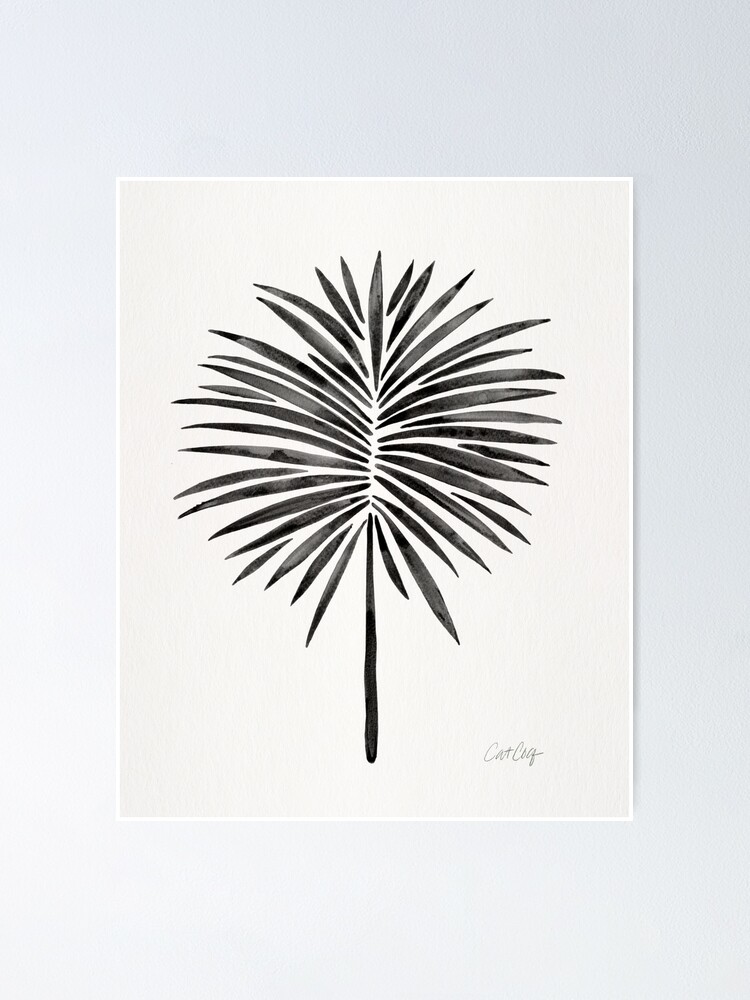The image is a black and white photograph taken indoors, displaying a rectangular piece of artwork mounted on a pale blue wall that fades to almost white in the lower left-hand corner. The artwork itself, framed by a thin white border, features a light gray background. At the center of this canvas, a plant or tree-like design is rendered primarily in black. The design consists of a thin vertical stem at the bottom, from which long, thin petals or leaves extend in a circular pattern around a central gap. In the lower right-hand corner of the artwork, there is a cursive signature that appears to spell out "CATCOG" or something similar in pencil. The photograph captures the image with clear clarity, under ample lighting, highlighting the simple yet intricate details of the artwork.